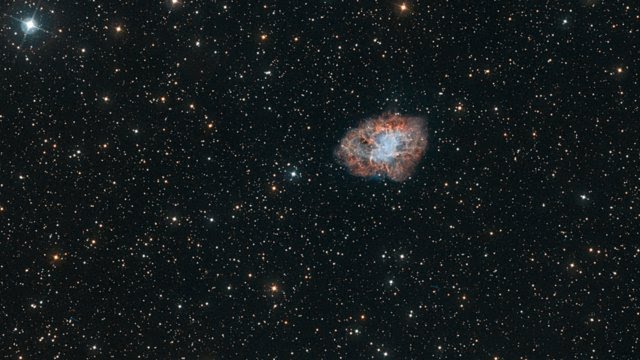The image captures a mesmerizing space photograph showcasing a distant star formation or nebula slightly off-center to the right. The nebula, resembling a loosely formed, irregular circle, possesses a captivating bluish-white core surrounded by wisps of reddish and tan gas, indicative of a celestial event or remnants of a stellar explosion. The background is predominantly black, dotted with numerous bright points representing stars or other galaxies of varying shades and intensities. Among this cosmic tapestry, a particularly prominent bright white star stands out in the upper left corner, noticeably larger and more luminous than the myriad of smaller stars scattered throughout the image. The stars vary in color from vibrant white to various tones of amber yellow, painting a vivid picture of the celestial skyscape.